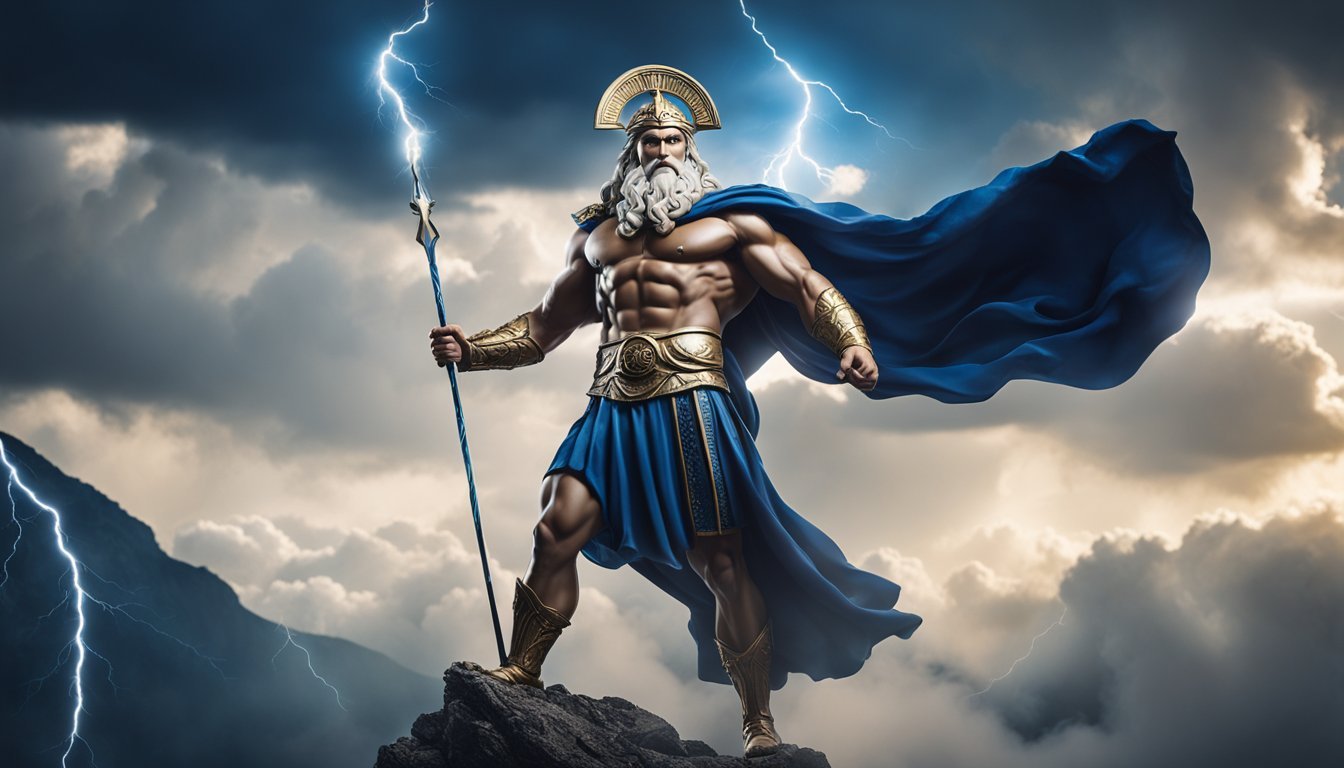This is a computer-generated image of a colossal, muscular Greek god, resembling either Zeus or Thor, standing majestically on the edge of a cliff. Towering and chiseled, he sports a thick, wavy white beard and long white hair, giving him a timeless, powerful presence. His intense, stoic gaze is directed into the camera, exuding an air of authority and warrior-like strength. Draped in a billowing blue cape, he wears a matching navy blue skirt, secured by an ornate, wide gold belt. Complementing his attire are gold boots, gold gauntlets, and a striking gold headpiece shaped like a half-moon or half-sun. In his hand, he holds a scepter or spear, from which bolts of lightning shoot out dramatically. The background depicts a stormy, tumultuous sky filled with dark clouds and frequent flashes of lightning, enhancing the god's powerful and commanding aura. A partial silhouette of another mountain is visible to the left, underscoring the dramatic setting of this divine and awe-inspiring scene.